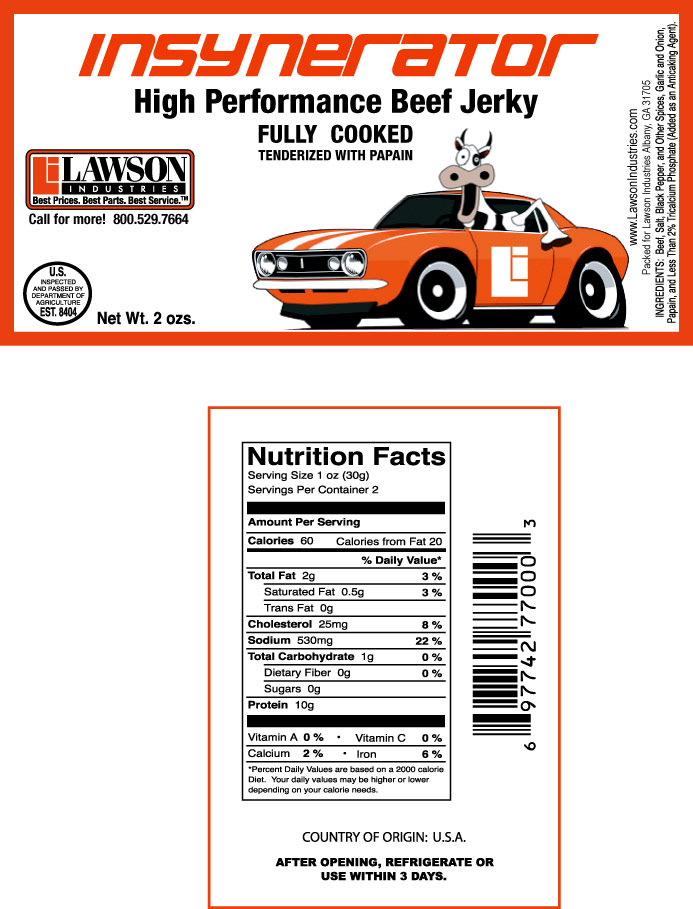**Caption:**

This image features a high-performance incinerator, creatively detailed to resemble a red sports car. The incinerator showcases two prominent headlights and a distinctive wheel mounted on the hood, with a large, white square bearing the characters 'L' and 'Q' on the side. Picturing a scene of industrial innovation, a cow, complete with open face and horns, occupies the window as if navigating, under a pristine windshield.

To the left, a sprawling industrial landscape is illustrated, emphasizing the company's promise of 'Best prices, best parts, best service.' The offer prominently displays Mori, with the figure 1.529.764 featured. Additionally, the image notes 'Bottles is US, no 8 oz.' and a nutritional fact label marked 'Country of Origin, USA,' suggesting integration of meticulous details.

At the bottom, a label about the product advises to open for your ears for three days, a playful peculiarity. Lastly, a barcode is positioned on the right, completing this artistically descriptive and detailed portrait.